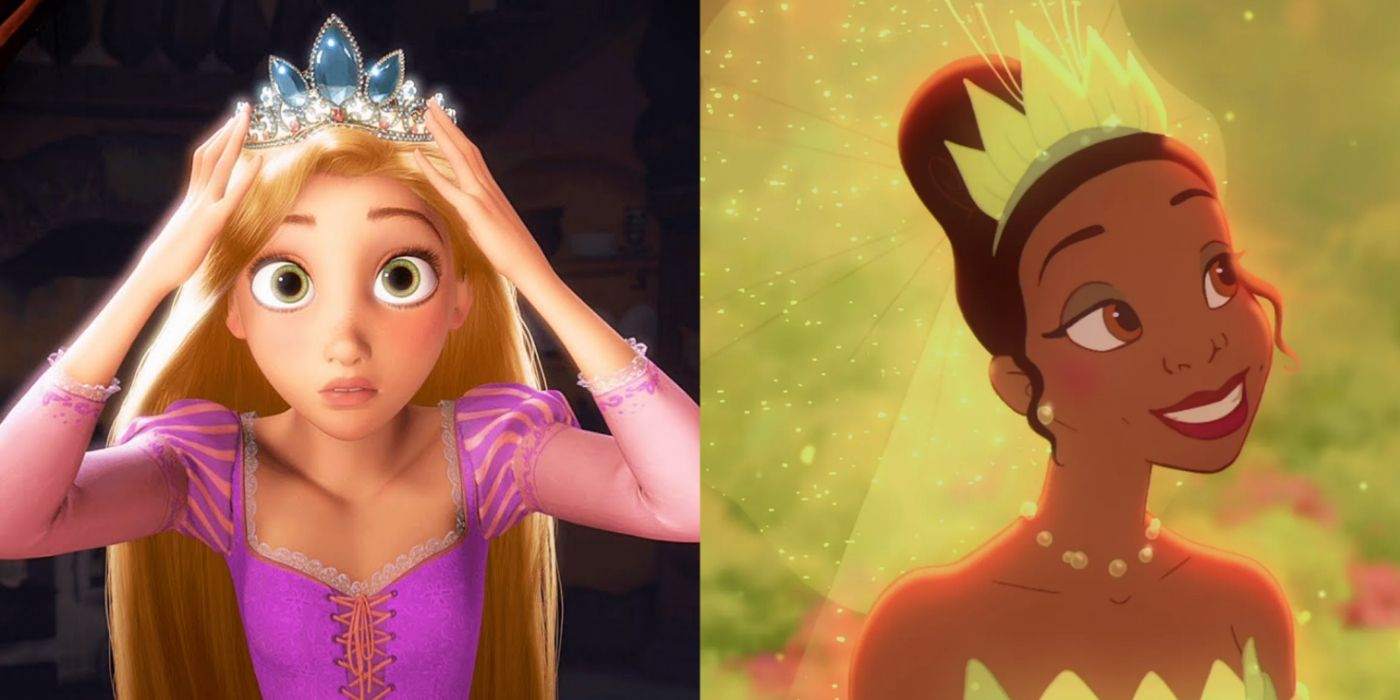In this photograph, two separate images feature characters from popular Disney animated films. On the left, we see Elsa from "Frozen" adorned in a detailed 1800s-style purple princess dress with a lace-up front and horizontal lace trim. Her short, puffy sleeves extend to see-through lace skin past her elbows. Elsa wears a crown embellished with three large jewels and several smaller ones, and her long blonde hair flows down, while her light green eyes and wide gaze are directed at the camera. She appears to be touching her crown with both hands.

To the right, we have Tiana from "The Princess and the Frog," set against a green backdrop. She is depicted facing slightly to the right and looking up, with a pleasant and content smile. Tiana wears a light green-yellowish crown that matches her necklace and bead earrings. Partially visible is the top of her dress, whereas a veil-like element can be seen behind her. The background suggests she is outdoors, with green flora and purple flower patches complementing the scene.